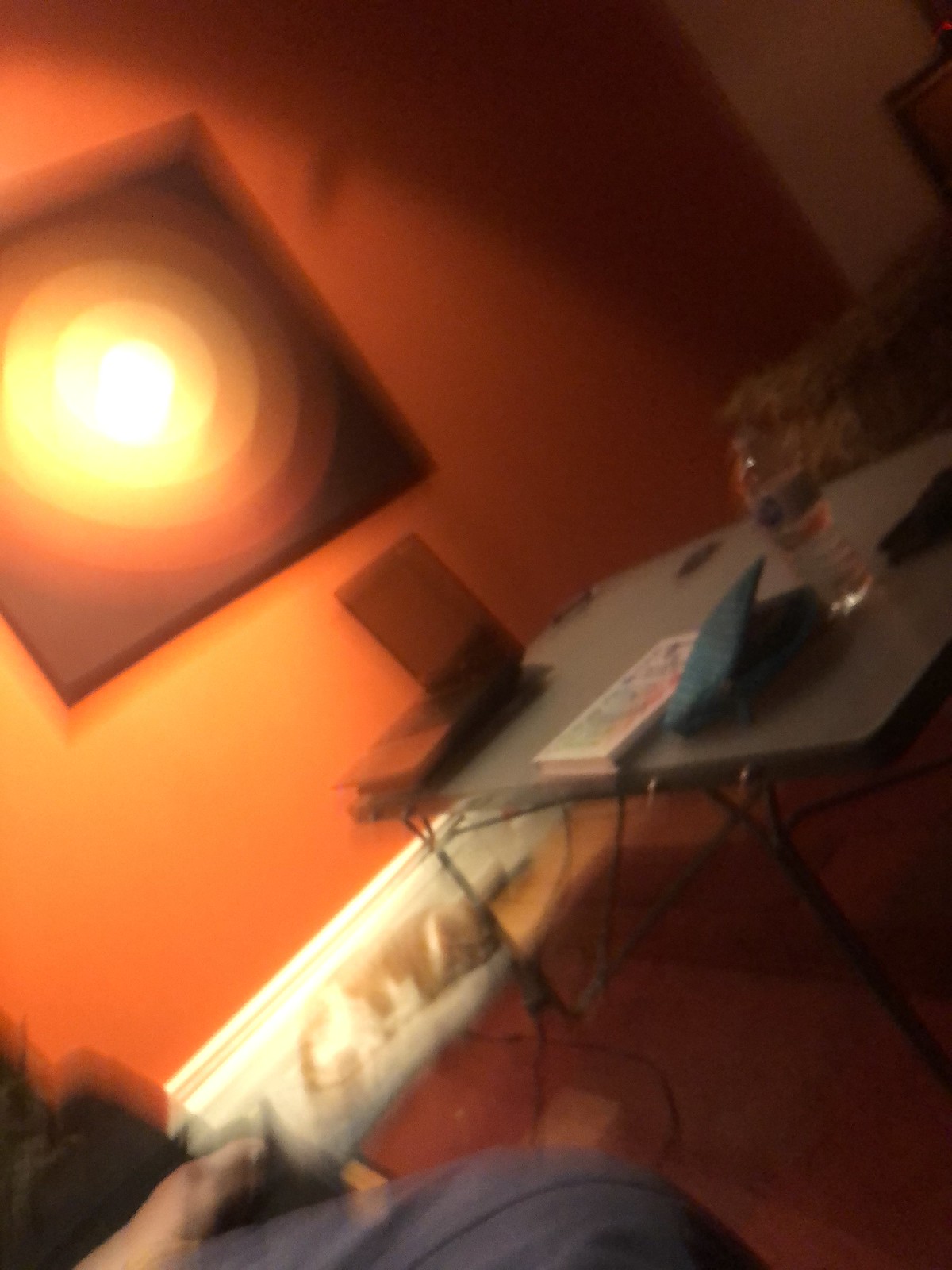A blurry, diagonally-taken photograph captures the cozy interior of a person's home. In the lower bottom left corner, a partial view of a person seated in a chair is visible; they are wearing a black shirt and gray pants, with an arm stretched towards the center of the image. The warm, orange-painted wall in the background is adorned with a white baseboard heater and a framed picture, most of which is visible except for its upper-left corner. The artwork features a series of small to large orange and yellow circles, all framed in dark brown. At the center of the scene stands a card table, upon which a laptop computer occupies the left-hand corner. Scattered across the table are several random items, including what appears to be a book, a phone, and a water bottle.